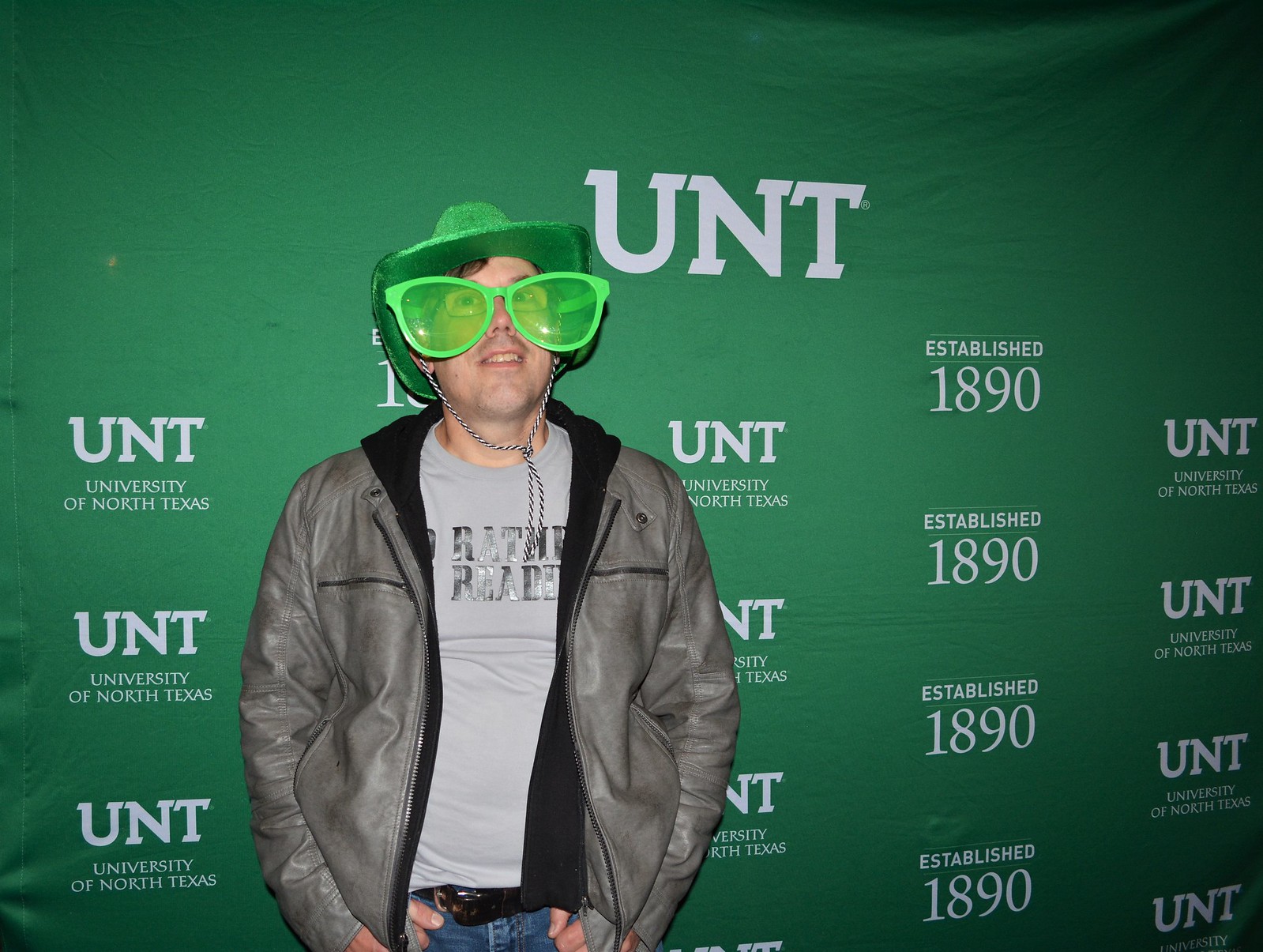The image captures a man posing for the camera against a backdrop promoting the University of North Texas. Centered slightly to the left, the man radiates a quirky charm in his eccentric outfit. He sports an oversized pair of lime green novelty sunglasses that sit hilariously over his regular glasses, and a matching green cowboy hat secured with a black and white string under his chin. His attire includes a gray leather jacket layered over a light gray t-shirt with partially obscured black serif text, and he pairs this with light blue jeans held up by a brown belt. Details of his surroundings reveal a green fabric backdrop emblazoned with repeated white text that reads "UNT University of North Texas Established 1890." The man, with a slightly awkward yet cheerful smile, appears to be participating in an event organized by the University.